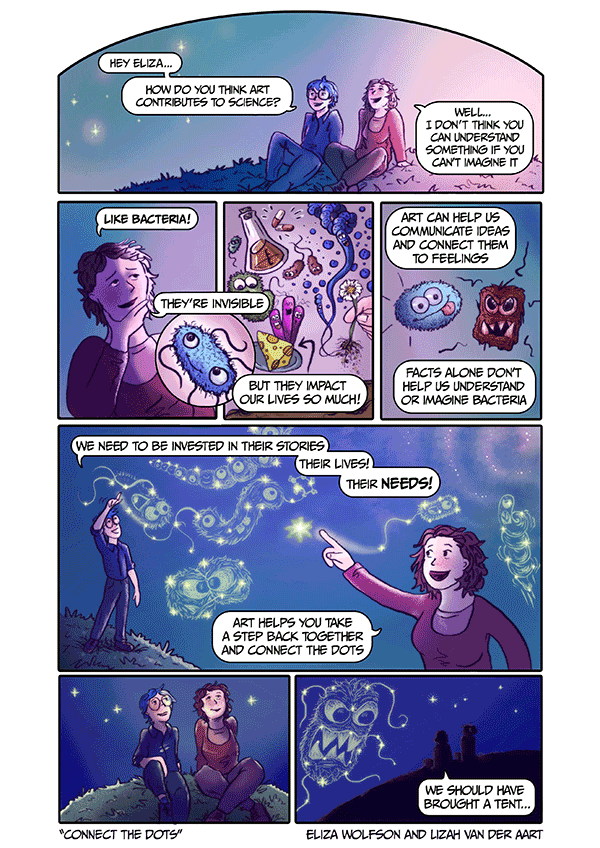A detailed comic strip with a predominantly blue-black background features seven cells, each contributing to a dialogue about the relationship between art and science. The strip begins with two people, one wearing a reddish outfit and the other in blue with circular glasses, sitting on a grassy hillside under a starry night sky. The conversation starts with, "Hey, Eliza, how do you think art contributes to science?" Eliza responds, "Well, I don't think you can understand something if you can't imagine it."

The next three cells zoom in on their dialogue. In the first cell, Eliza explains, "Like bacteria, they're invisible but they impact our lives so much." The middle cell depicts various bacteria—squiggly figures with faces—saying, "Art can help us communicate ideas and connect them to feelings." The dialogue elaborates, "Facts alone don't help us understand or imagine bacteria." The third cell continues, emphasizing the narrative and emotional connection art provides.

Beneath these, a larger panel shows the pair standing on the hillside with stars twinkling around them, continuing the conversation about the importance of art in understanding science. The final cells return to the two people now darkened, still on the hill, looking at the night sky. They see constellations in the form of monsters and bacteria, leading one to say, "We should have brought a tent."

The bottom of the strip features the title "Connect the Dots," with stars intricately outlined in white, and credits "Eliza Wolfson and Lisa Vander Art" on the lower right-hand corner.